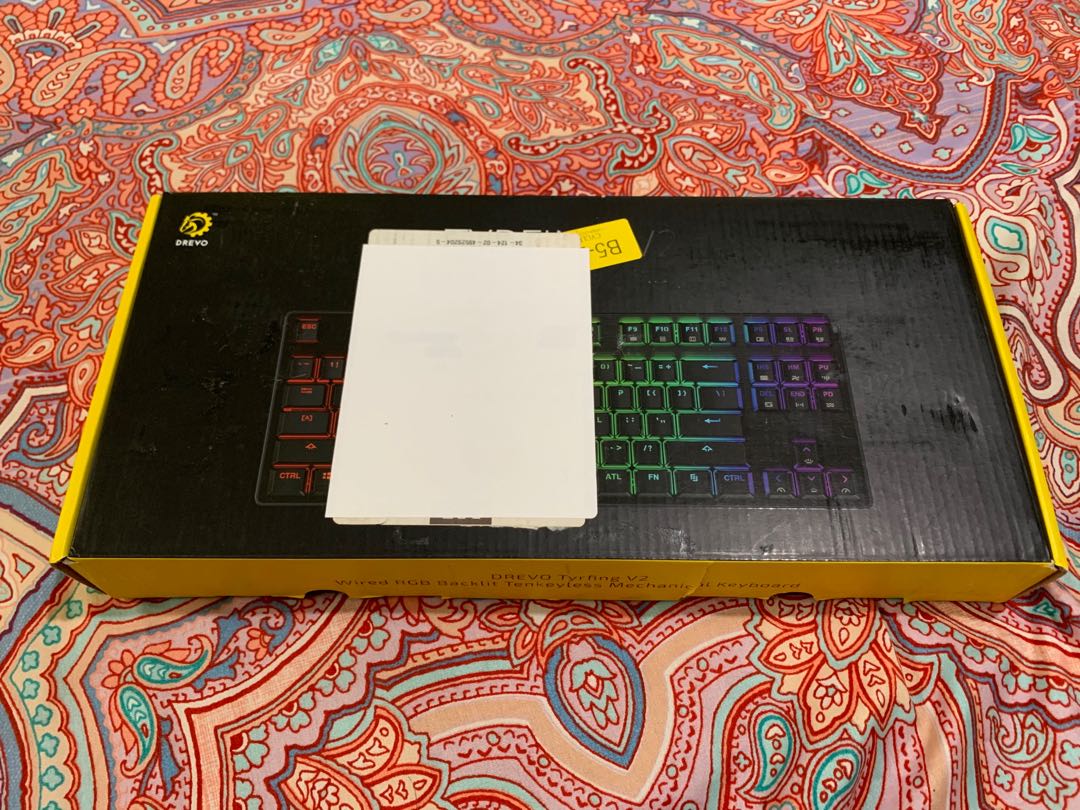The image showcases a Drivo (or Drevo) branded keyboard, specifically identified as the "TYRFING V2." This wired, RGB backlit, tenkeyless mechanical keyboard is presented in its original packaging. The box's design features a black lid with yellow edges, and a prominent yellow section on the front where the brand name and product details are displayed in black text. The keyboard itself is depicted in black within the box, adorned with a white sticker on the left and another gold or yellow sticker beneath it. Surrounding the box is a vividly colorful blanket or sheet, blending hues of red, blue, violet, pink, green, and peach, adding a striking contrast to the packaging. The box also displays a rainbow RGB effect behind the illustrated keys, highlighting one of the keyboard's key features.